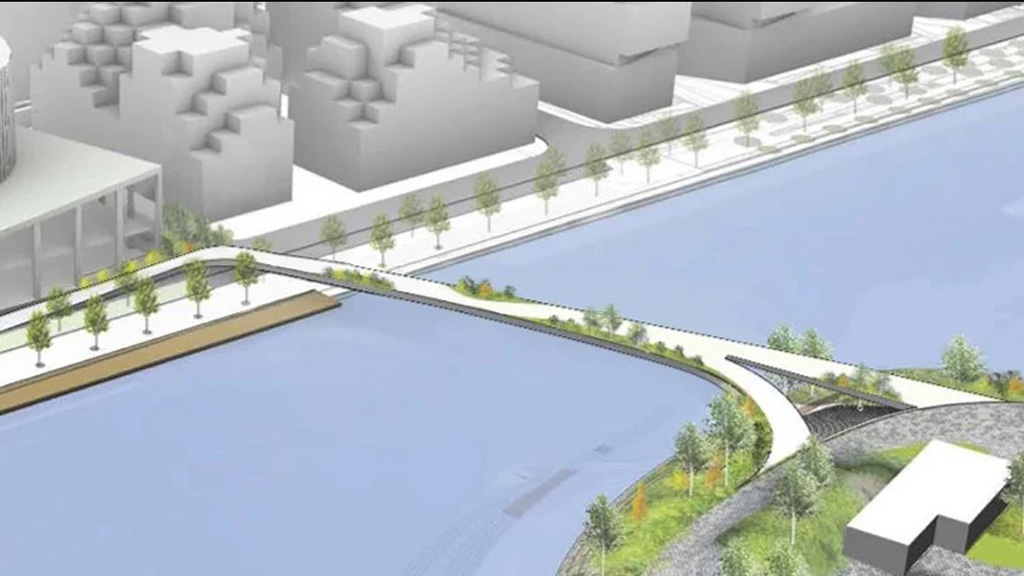The animated image, resembling graphics from a video game or an older edition of Google Earth, depicts a 3D-rendered bridge stretching across a body of water with blue hues. This thin bridge, populated with lush green foliage, may serve as a pedestrian walkway rather than being for vehicle traffic, owing to the natural growth along its span. The bridge connects two distinct areas: on one side, there are towering buildings and a paved water walkway, while the opposite side features an area with smaller, one-story buildings and a dock. The surroundings on either side of the bridge include incomplete block-like buildings and clusters of trees. Notably, the bridge's structure steps down toward the lower left where several paved walkways and a gray-walled building with a white roof are situated on a round piece of land. The bridge, replete with its natural and constructed elements, seems to harmoniously link the two diverse landscapes.